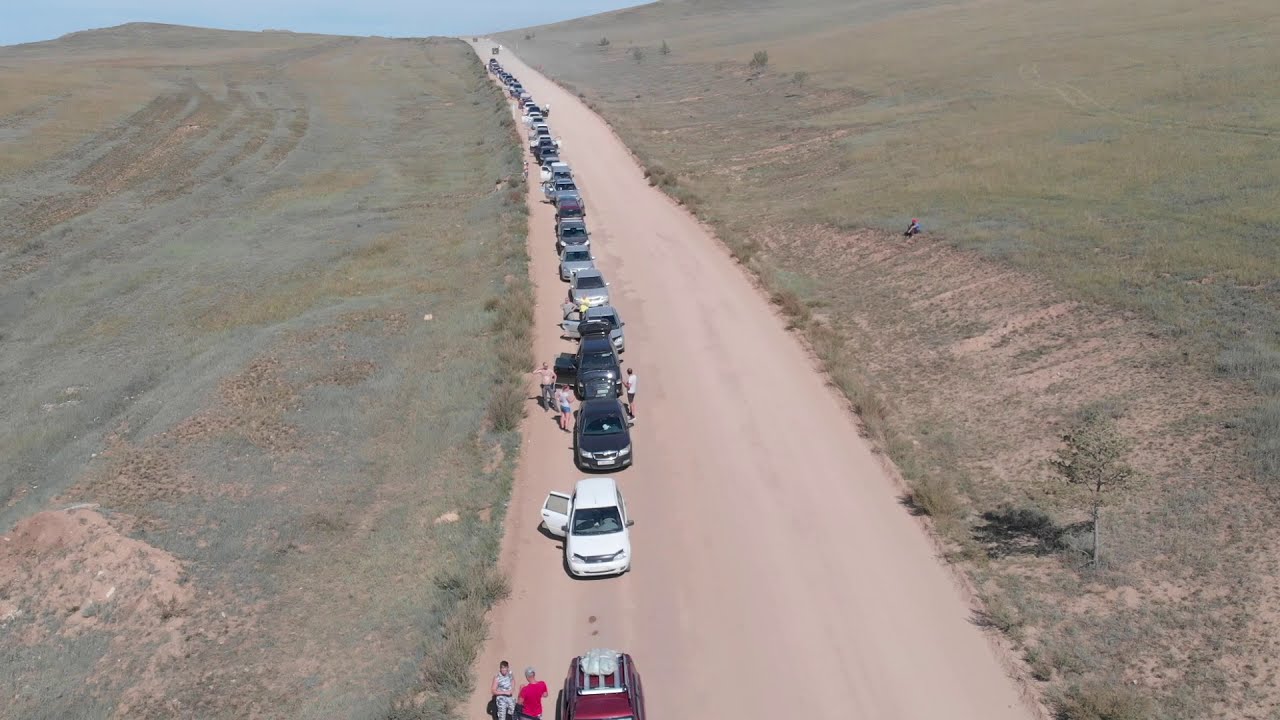The photograph, taken outdoors during the day, captures a long dirt road stretching from the bottom center of the image all the way into the distant background. The road is flanked by expansive fields of green grass interspersed with patches of dry, brown or yellow areas, creating a vivid natural setting. On the left side of the road, a continuous line of cars extends from the foreground deep into the background, featuring a diverse assortment of colors including red, white, black, silver, and gray. In the very foreground, a red car is prominently positioned with two individuals nearby—one in a red t-shirt facing away from the camera, and another person in a black and white or gray and white outfit gazing directly at the camera. Adjacent to them is a white vehicle with its passenger door open, followed by two black vehicles and several more cars further down the line, some with doors open. Additionally, scattered around these vehicles are people standing or sitting, including one individual seated on a slight incline on the right side of the road, gazing down at the scene. The landscape includes a single tall tree and some bushes and hedgerows alongside the dirt road, enhancing the outdoor ambiance of the photograph.